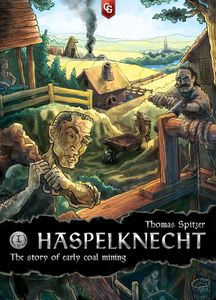This cover features an illustration that vividly depicts a rustic early coal mining camp set against a backdrop of a blue sky and expansive green field, dotted with houses, huts, and trees. The houses are reinforced with wooden planks acting as barricades and have chimneys emitting black smoke. The scene is bustling with activity: a man turns a wooden crank, possibly lowering a bucket into a mine pit, another man pushes a cart, one draws water from a well, and another carries items on his shoulder. Above this detailed tableau, in the upper left corner, is a small silver circle with an eye in it. The book’s title, "Thomas Spitzer: The Story of Early Coal Mining," is prominently displayed in silver text on a black background at the bottom of the cover.